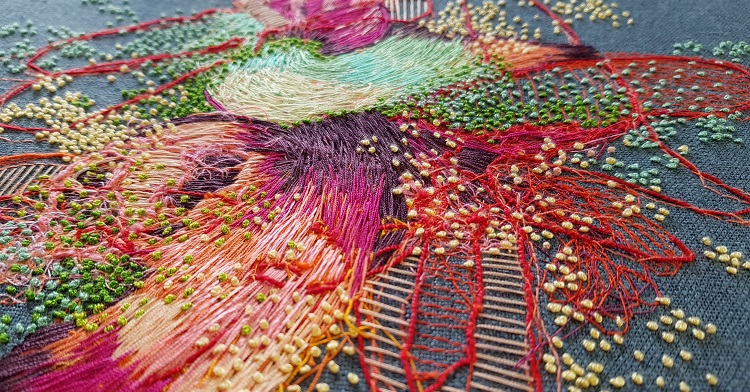This image showcases an intricate piece of modern textile art on a bluish-gray, loosely knit or denim-like canvas. The artwork is crafted primarily using embroidery threads in a vibrant color palette, including deep blues and whites, verdant greens, and fiery reds that outline shapes reminiscent of butterfly wings. Interspersed with these motifs are sweeping threads in purples, pinks, oranges, and yellows, contributing to the dynamic and colorful composition.

The focal point appears to be an abstract representation of a postmodern flower, featuring a circular form with a central point at the top and a long, rainbow-colored, stem-like shape extending downwards, framed by broad, abstract petals. Intricate French knots punctuate the fabric, creating textured dots in creams, greens, turquoise blues, and lighter blues. These knots scatter across the textile, adding depth and a touch of whimsy to the vibrant tapestry. The meticulous needle-pointing highlights details such as saffron flowers with golden petal dust and additional red and green floral elements, showcasing the artist's dedication and skill. This fusion of colors, textures, and forms results in a stunning, richly detailed textile painting.